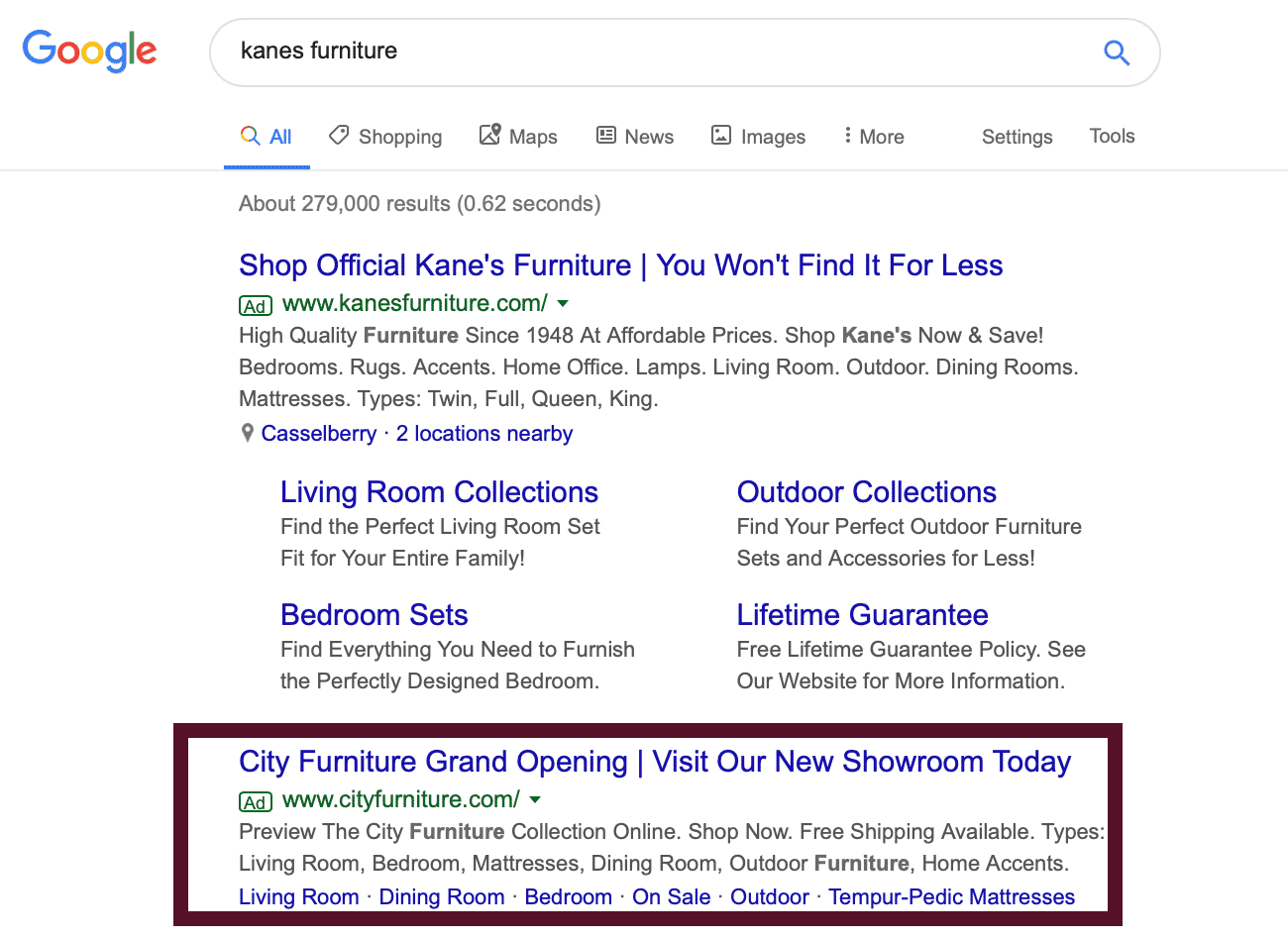The image depicts the results of a Google search for Cane's Furniture, a furniture company with the tagline, "You won't find it for less." The search results page is prominently displayed, and one particular result stands out. Highlighted with a burgundy rectangle is a listing for City Furniture's Grand Opening, which may be a competing furniture store. The emphasis on this result suggests a potential rivalry or significant event. The search offers no additional information about Cane's Furniture, leaving the user unsure about the company's quality or reputation.